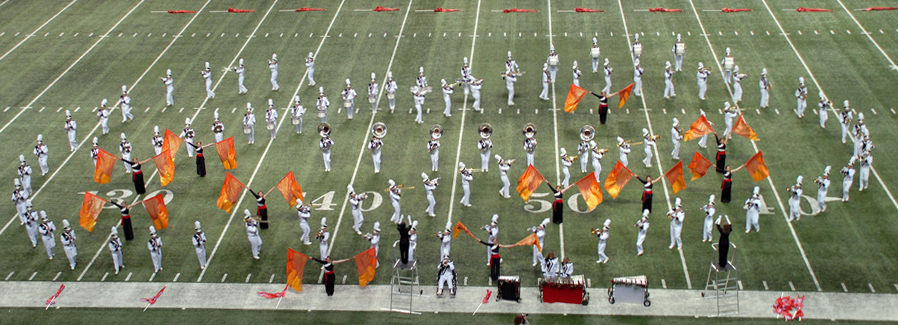This photograph captures a detailed scene of a marching band performing on a green grass football field, likely during a halftime show. The entire band is dressed in striking white uniforms, adorned with large white feathers on their caps, which provide a unified and imposing visual display. Positioned near the midfield, around the 50-yard line, the band members are arranged in a precise formation resembling interlocking loops. Central to the formation are the brass tuba players, surrounded by musicians playing smaller horn instruments. Among the performers, there are individuals in black, white, and red uniforms energetically holding large orange and red flags, potentially cheerleaders or spirit leaders, adding vibrant splashes of color to the scene. The band appears stationary, with some musicians in the front holding two orange flags and others playing big horns. The scene exudes a sense of coordinated order and spirited performance. Although there is no date or identifying text, the image likely represents a university due to the style and coloration of the uniforms.